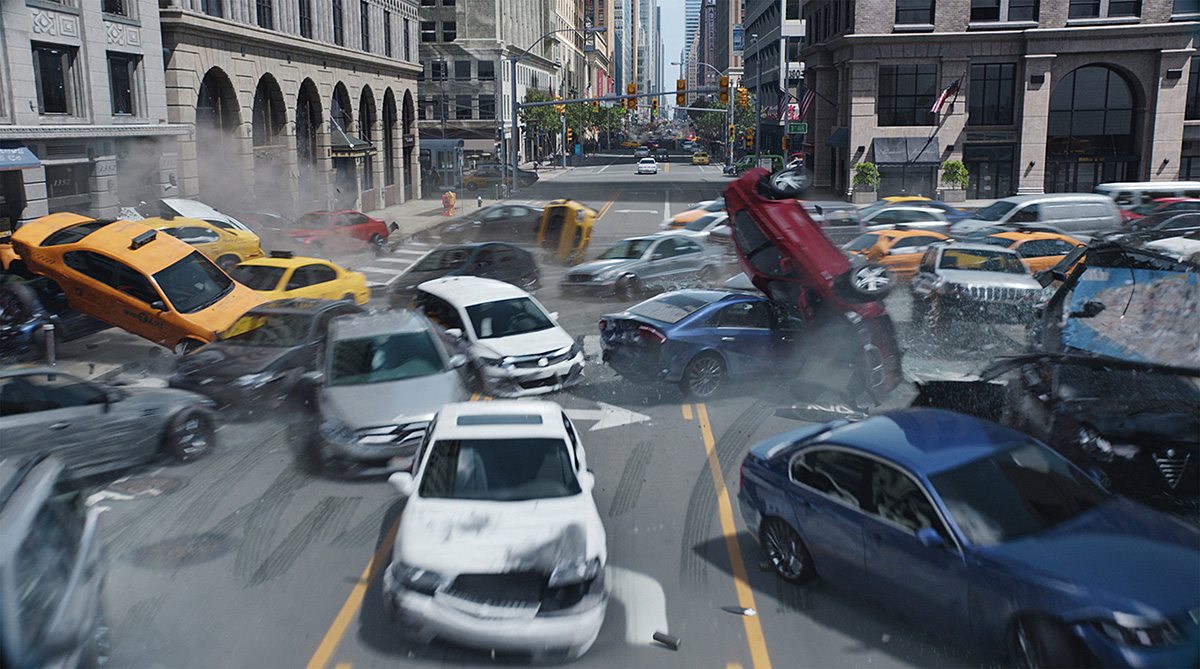The image depicts a chaotic and massive car crash in a dense urban area, likely a scene designed for a movie given the scale of destruction and absence of people. The crash involves about 15 to 20 vehicles, including yellow taxis, minivans, sedans, SUVs, and a possible car hauling truck. Some cars are flipped over or stacked upon each other precariously. In the foreground, a white four-door car has a damaged front right side, while to its right, a burgundy car is tipped over, leaning on a navy blue car. The scene is set in a bustling downtown area with multiple lanes, formal-looking multi-story buildings, and high-rises, possibly in cities like Boston or San Francisco. Office buildings adorned with American flags and distinctive arches frame the streets in the background, and there are concrete buildings with speakers. The photograph is taken during the daytime, highlighted by sunlight and some clouds in the sky, indicating a street filled with chaos and destruction, yet with untouched surrounding buildings, emphasizing the dramatic aftermath of the incident.